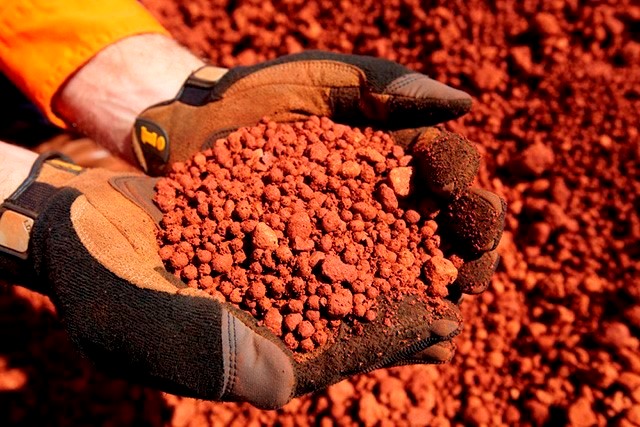In this photograph, two gloved hands prominently hold a large quantity of vibrant red-orange, pebble-sized granular substance. The coarse material fills both the cupped hands and the entire background, suggesting a vast expanse or container of the same reddish rocks or gravel. The gloves, appearing sturdy and suitable for work, are distinctively colored with orange palms, black backing, and brown accents, and they fit snugly around the wrists. The extended hands, likely of a white male, emerge from yellow sleeves. The overall composition is strikingly dominated by the red-orange hue, casting a warm reflective glow on the person's light skin, accentuating the uniformity and texture of the scene.